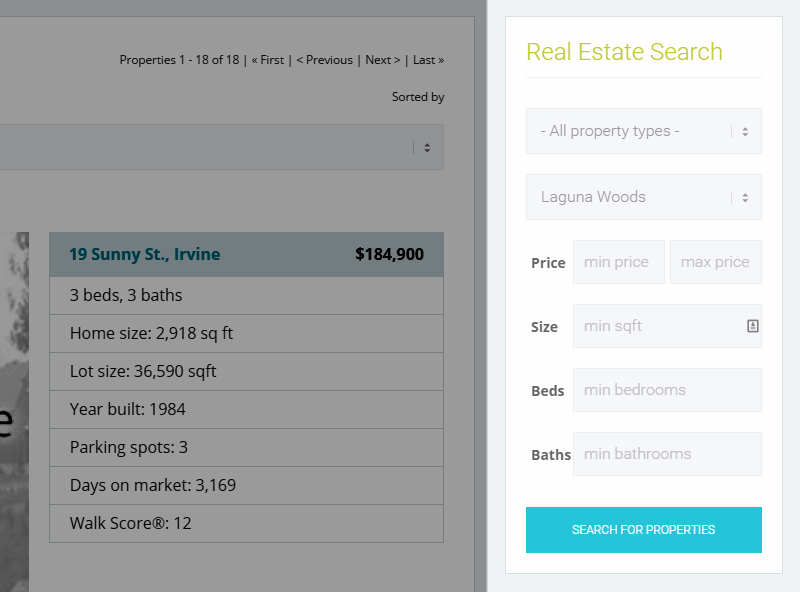This screenshot captures a detailed view of a real estate search interface. On the right side, several filters and options are displayed prominently, including a drop-down menu for "All Property Types" and another for selecting locations, with "Laguna Woods" currently chosen as the location. The interface allows users to set parameters such as minimum and maximum price, minimum square feet, minimum number of bedrooms, and minimum number of bathrooms. 

A notable section of the interface is highlighted, showing details of a specific property at "19 Sunny Street, Irvine." Listed for $184,900, this property features three bedrooms and three baths, with a home size of 2,918 square feet and a lot size of 36,590 square feet. Built in 1984, it includes three parking spots. The property has been on the market for an impressive 3,169 days. 

Additionally, the interface provides a "Walk Score" of 12, suggesting that the location may not be very pedestrian-friendly and residents might need to rely on cars for daily errands. 

A blue "Search for Properties" button with white text is situated at the bottom of the filter options. The background displays a list of 18 properties returned by the search, though only the text details of the highlighted property are fully visible, with no image shown. The interface also allows for sorting by different filters to refine the search results.